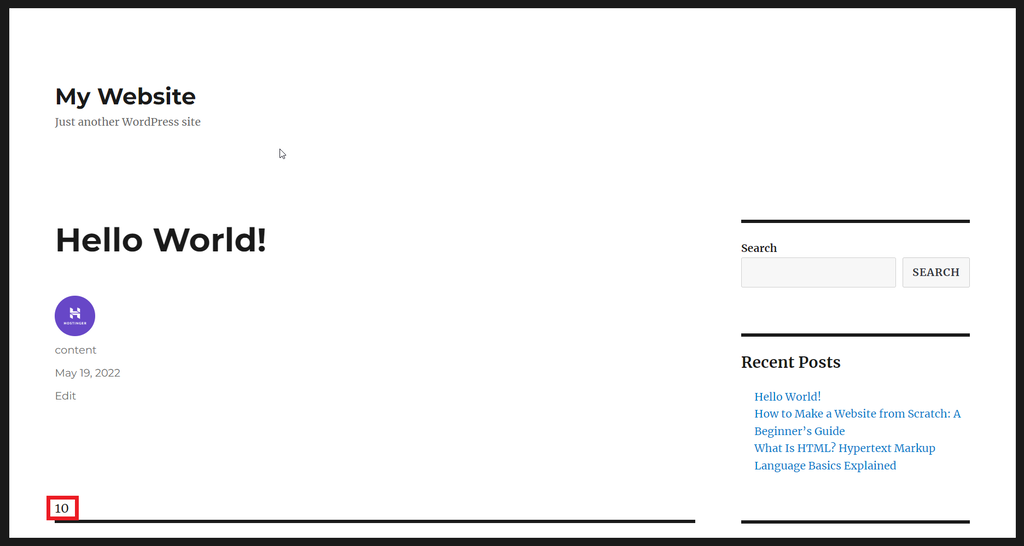The image showcases a minimalist web page with distinct sections:

1. **Header**: Framed within a white box with a black border on all sides, the top left corner prominently features "My Website" in bold black letters. Directly beneath in small gray font, it reads "Just another WordPress site."

2. **Main Content**: Centered below the header, the phrase "Hello World" is displayed in large, bold black letters, marking the introductory content. Just below, there's a timestamp stating "Content: May 19, 2022," followed by an "Edit" option. A purple circle is situated beneath this text.

3. **Separator and Metadata**: A black horizontal line runs across the page's width, breaking up the sections. To the left of this line, the number "10" is encased in a red box.

4. **Search Feature**: On the right side of the page below the black line is a search bar, with the word "Search" below it. The search bar itself has a gray "Search" button on its right.

5. **Recent Posts**: Another black horizontal line demarcates the start of the "Recent Posts" section. Listed under this heading are several blue hyperlinks:
    - "Hello World"
    - "How to Make a Website from Scratch: Beginner's Guide"
    - "What is HTML? Hypertext Markup Language Basics Explained"